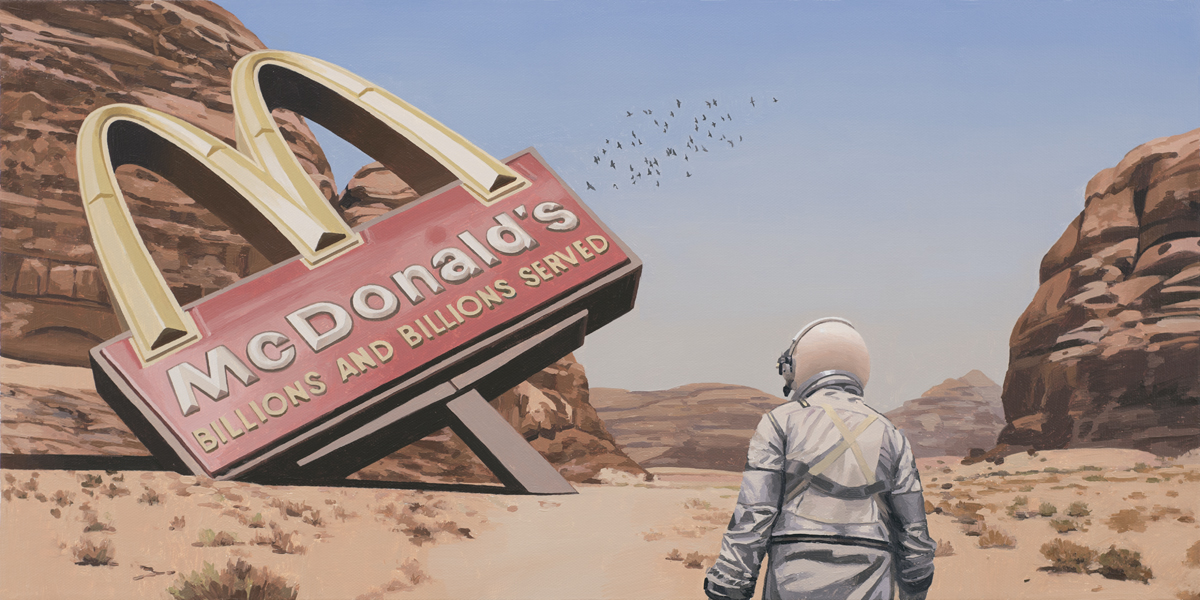In this surrealist-style illustration, a person clad in a retro sci-fi, silvery satiny jacket and a white helmet stands in the foreground, facing a barren desert landscape reminiscent of Arizona or New Mexico. The desert scene unfolds with sand-colored terrain punctuated by small brown shrubs and numerous rocky formations, including modest mountains and plateaus. The sky transitions from beige at the horizon to clear blue at the top, with a hazy quality in the distance that gently obscures the farther rocky structures. A notable feature is a tilted, partially fallen McDonald's sign leaning against a prominent rocky formation on the left. The iconic golden arches and red rectangle adorned with the text "McDonald's" and "billions and billions served" stand out in bold white and yellow fonts, adding a touch of commercial nostalgia to the scene. In the distance, a flock of small black birds punctuates the sky, emphasizing the desolation and expansive scope of the landscape.